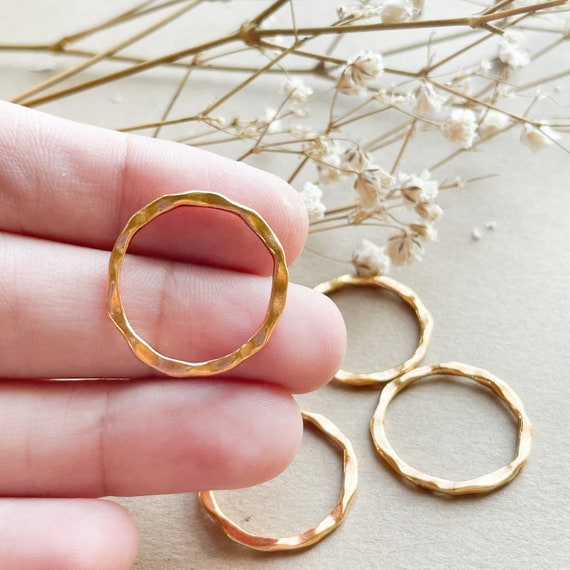The image features a close-up of a hand emerging from the left side, its four fingers partially visible with a gold ring resting on the top two fingers. The ring has a distinctive ridged texture along its center. The hand is positioned over an off-white surface, which also displays three additional gold rings, each identical in their ridged design. Above these rings lies a delicate arrangement of dried white flowers, possibly resembling baby's breath, attached to slender brown branches. The flowers and branches extend toward the upper section of the image, providing a soft, decorative backdrop that enhances the visual appeal of the gold rings.